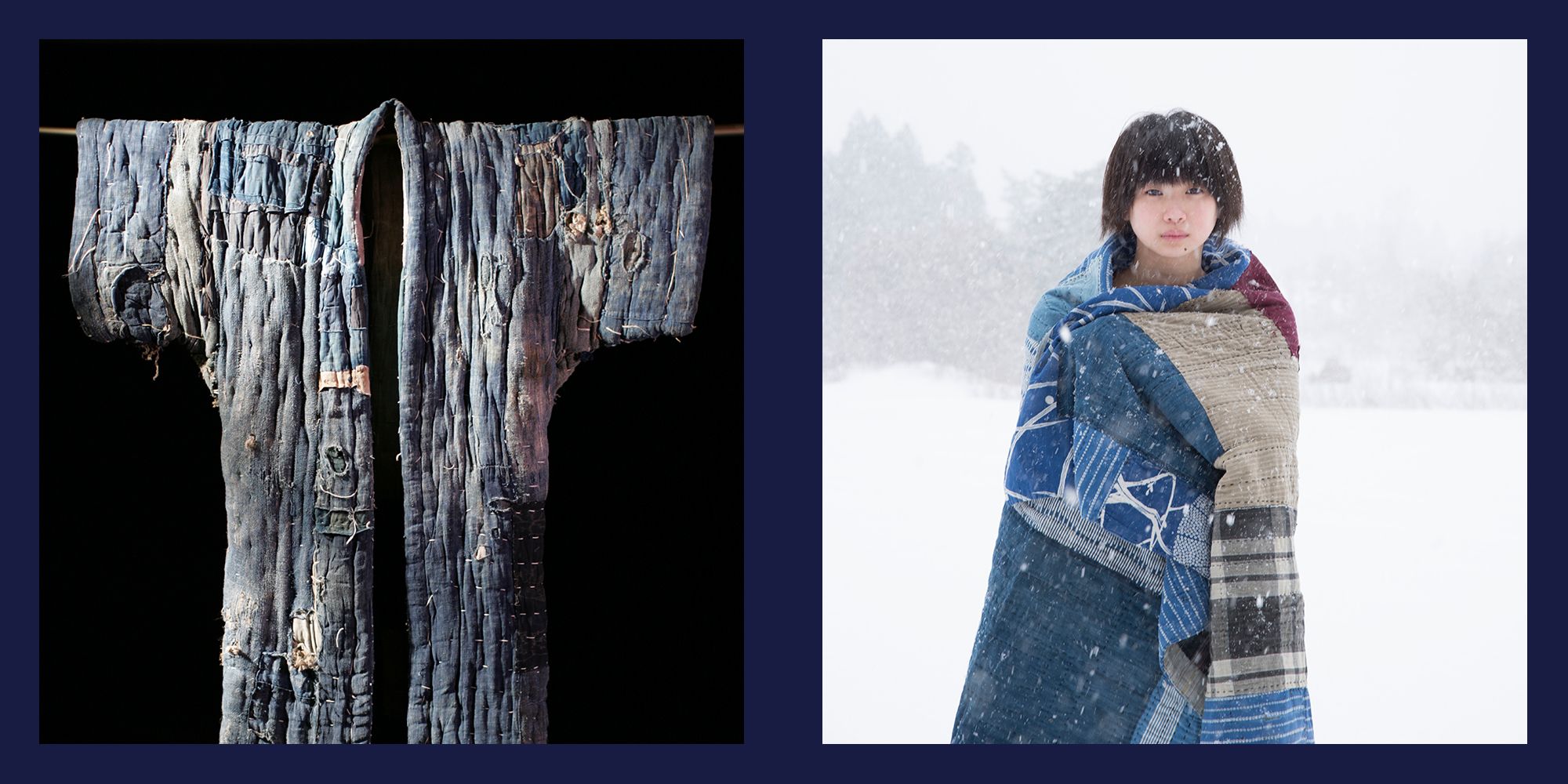This landscape image, framed by a navy blue border with a vertical divider in the middle, showcases two complementary halves. On the left, a black background sets the stage for a textured patchwork piece crafted from various fabrics, predominantly jean material. The assembly, resembling an oversized, ill-fitting coat or blanket, features uneven stitching and alternating fabric colors, creating a visually intriguing garment.

In the right half of the image, an Asian individual with a mushroom bowl cut hairstyle stands against a bright, snowy backdrop that almost obscures the tree line. The snowy setting, detailing snowflakes delicately settled in the person's hair, enhances the cold atmosphere. This individual is wrapped in a quilt-like covering composed of different fabric sections, with dominant shades of blue interspersed with other colors like brown and red. This quilt provides a visual connection to the patchwork on the left, suggesting that the garment they are wearing is the same as the textile piece depicted on the opposite side. The day-time setting adds a serene brightness to the snowy scene.